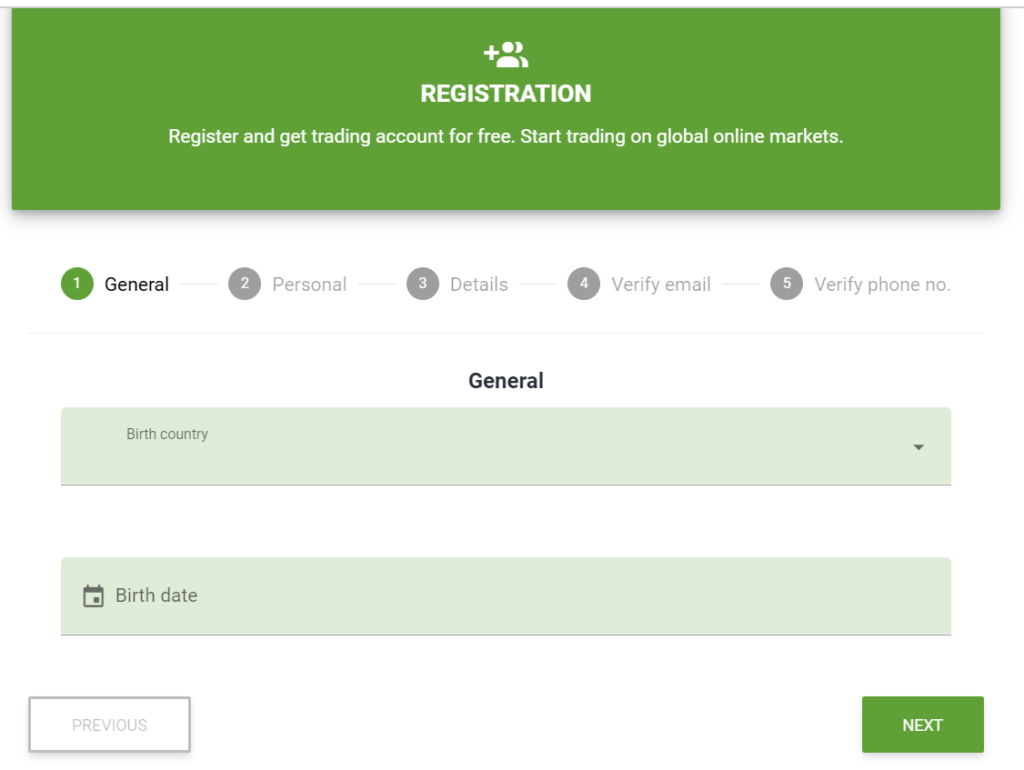This screenshot, likely taken from a computer screen due to its wide aspect ratio, displays a registration page for a trading platform. The upper section of the screen features a large, green rectangle that spans the width of the page. Centrally positioned within this green banner is a plus sign flanked by two outlined figures, with the word "Registration" written in white directly below it. An accompanying text below this header reads, "Register and get a trading account for free. Start trading on global online markets," all meticulously centered within the green rectangle.

Below this introductory section are five sequential registration steps, each represented by a grey circle with corresponding labels: 
1. General (highlighted and active in green)
2. Personal
3. Details
4. Verify Email
5. Verify Phone Number

These circles are arranged horizontally, and only the first step, labeled "General", is in a highlighted green circle indicating it is the current step. The remaining steps are greyed out, signaling that they have not yet been completed.

Underneath this steps indicator, the section for "General" is displayed. It contains fields for "Birth Country" with a dropdown menu, and "Birth Date", which also appears as a dropdown menu selection rather than a text input. These input fields are presented in a lighter green color, contrasting with the overall white background of the page. The darker green color used at the top for the banner and the number "1" circle is visually matched to tie the design together.